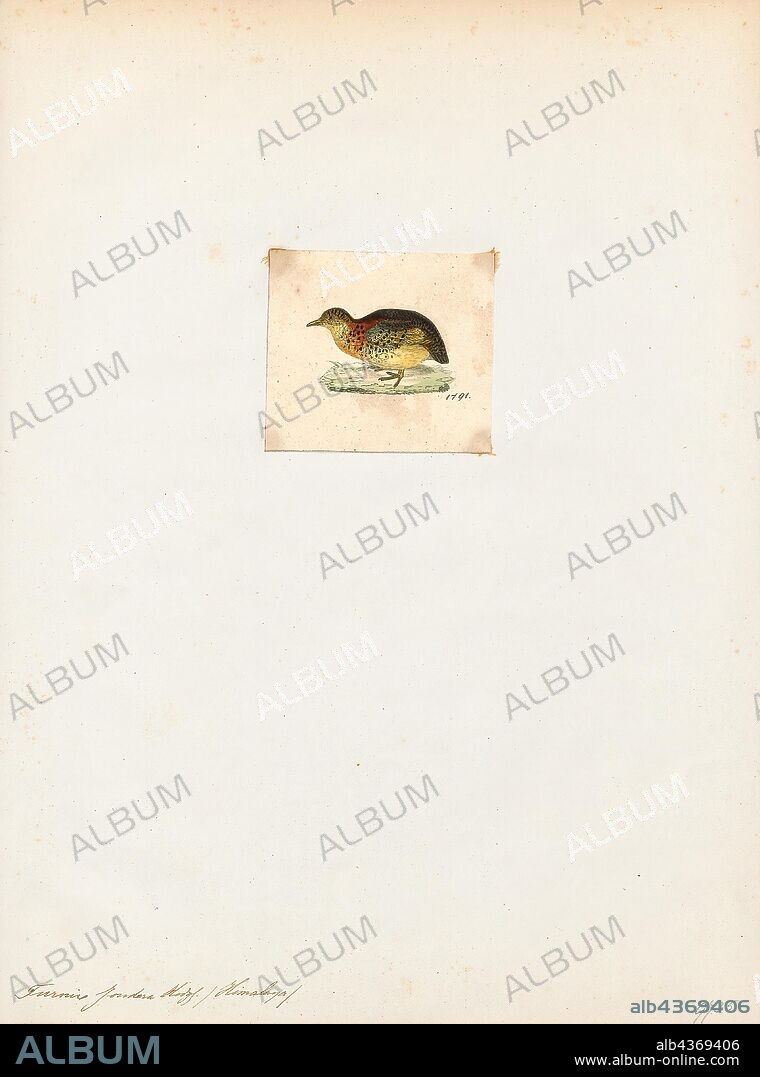This image showcases a detailed pencil and colored pencil sketch of a small bird, possibly a quail or similar ground bird. The bird stands on a greenish patch of grass or a wooden plank, facing to the left. Its head is yellow, adorned with small black dots, and its underbelly shares the same yellow hue. The bird's neck and chest display a reddish collar with black spots, while its back and tail are darker, shaded with grey or black tones. Its wings are yellow, also highlighted with black spots, and it has a three-toed foot. 

The artwork is presented on a small square canvas, placed against a larger off-white rectangular background. This background features the watermark “ALBUM” repeatedly in gray and white, arranged diagonally across the image. At the bottom of the image, there is a black bar with the word "ALBUM" in teal and grey text, along with the web address “www.album-online.com” and the identifier “ALB4369406”. Above this black bar, to the left, there is an author’s signature, which is too small to read.